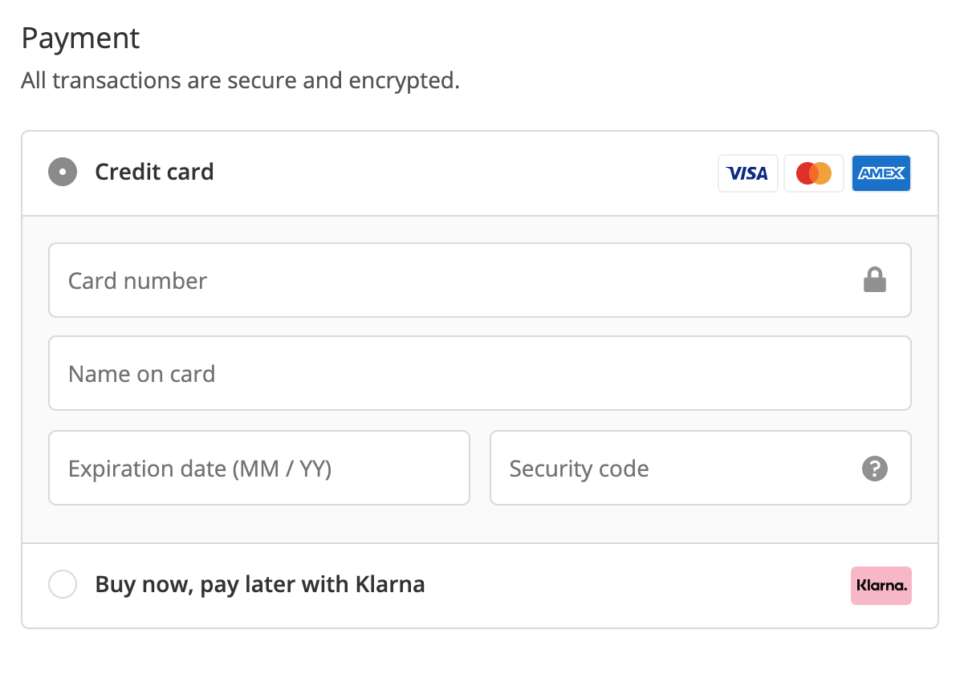Screenshot of a Payment Section

The image displays an online payment interface set against a white background with a gray border around the main section. The header informs users that "All transactions are secure and encrypted."

Underneath, the "Credit Card" payment option is selected, and icons for Visa, MasterCard, and American Express (Amex) are visible. Below these icons, there is a field for entering the card number, accompanied by a lock icon, which signifies security.

Further down, fields for the "Name on Card," "Expiration Date" (formatted as two digits for the month and two digits for the year), and "Security Code" are present. A question mark icon next to the "Security Code" field likely offers additional information on what the security code is.

Additionally, there is an option for "Buy Now, Pay Later with Klarna," though the credit card option is currently selected. No information has been entered into any fields.